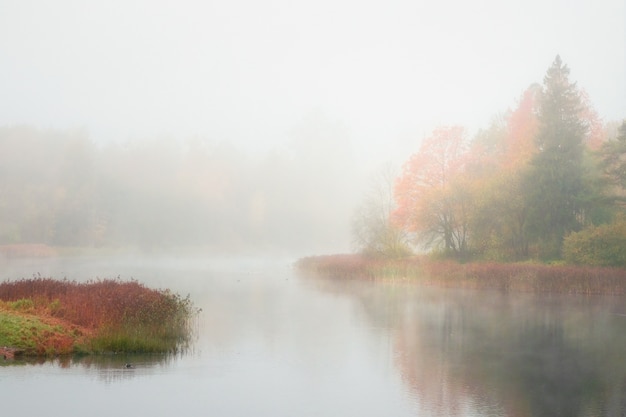This image depicts a captivating landscape scene featuring a serene lake or river, with a small island at its center adorned with vibrant, reddish-pink vegetation. Surrounding the water, the banks are lined with similar brightly colored flora, interspersed with tall green weeds and grasses. There are various types of trees growing along the shores, including pine trees and deciduous trees showing the classic colors of fall. The scene is enveloped in a dense fog, giving the entire picture a hazy, mystical quality. Silhouette-like trees can be seen on the left side of the water, their reflections shimmering on the calm surface. An additional tree line in the background further fades into the mist, suggesting an early morning setting bathed in soft daylight. The overall atmosphere is tranquil and ethereal, blurring the lines between reality and artistry.